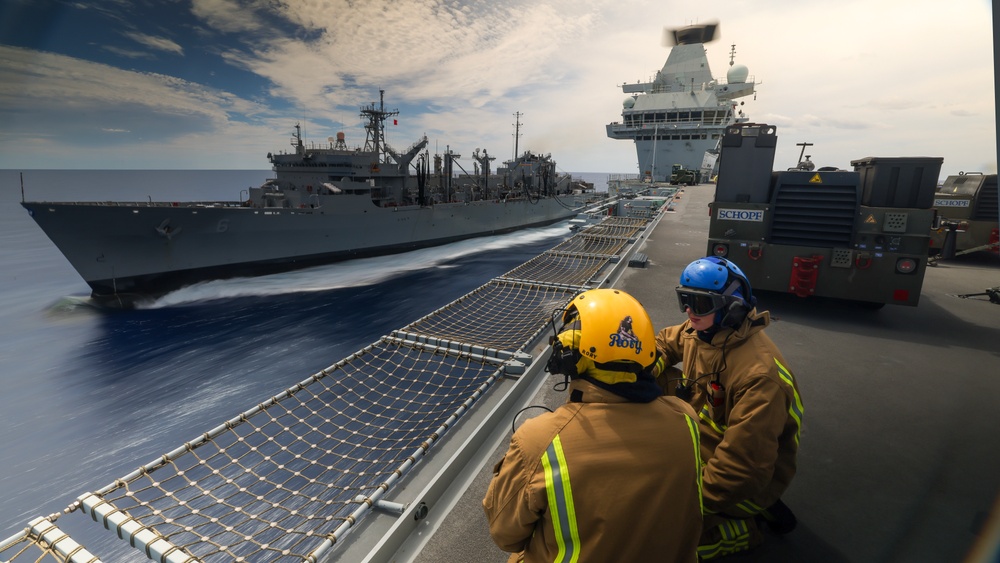This detailed color photograph captures a serene maritime scene featuring two military vessels—the foreground showcases an aircraft carrier with distinctive details, while a destroyer sits nearby in the calm blue ocean. The photograph is wide and horizontal, providing a panoramic view of the scene under a blue sky strewn with white streaks of clouds. On the deck of the aircraft carrier, two individuals are visible; both are wearing light brown jumpsuits with green safety stripes, along with dark goggles and headphones. One wears a yellow helmet, and the other a blue helmet. The waist-up view of these figures highlights their safety gear and attire. The aircraft carrier is lined with netting above the water's edge, adding an element of preparedness and security. In the background, the control tower crowned with a radar stands prominently. Adjacent to the aircraft carrier, the light-colored steel destroyer, characterized by its rectangular shape with pointed ends, sits closely. The destroyer features several towers, including one with radar equipment, and has a large truck marked with blue lettering that reads "SHOPE" on its deck.